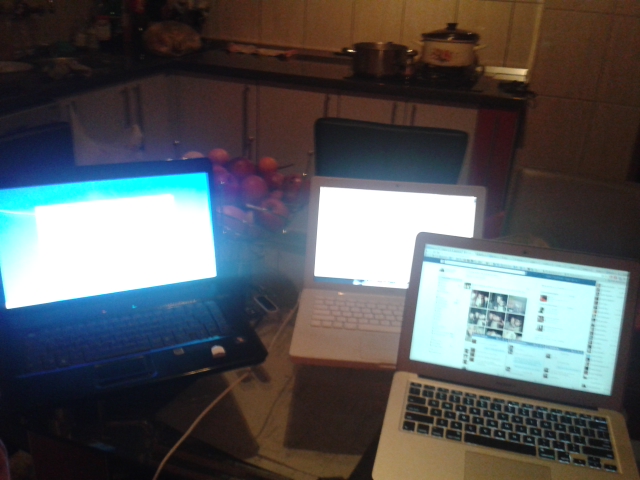The photograph captures a scene of three laptops arranged on what appears to be a kitchen table, situated in a dimly lit room, possibly indicating the setting is a personal home. In the foreground to the right, there's a modern gray or white MacBook with black keys, visibly displaying Facebook. To its left, partially obscured, is another laptop, an older all-white MacBook, with a screen emanating a bright white light. The third laptop on the far left is black with black keys, showing a bright blue screen with a white rectangle in the middle, likely a PC rather than an Apple product. The table they rest on is suggested to be made of glass due to visible reflections and shadows beneath the devices. A bowl of assorted fruit, prominently featuring apples of various red shades, sits behind the laptops, along with kitchen countertops adorned with crockpots, cooking pots, and cutlery, subtly visible in the background.